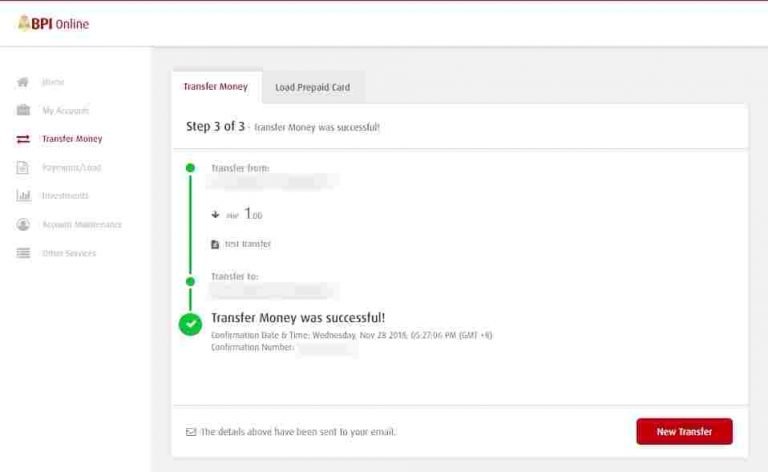A screen capture of a website window labeled "BPI Online" in maroon-colored font. To the left of this label is an indistinct, off-color greenish-tan logo. At the very top of the image is a thin maroon line. The left-hand side of the page features a navigation pane on a white background, under the BPI Online header. The top icon in the navigation pane appears to depict a house, though it's blurry and illegible; next to it is a vague label. Beneath that is a gray square labeled "My Accounts." Further down is a maroon-colored tab titled "Transfer Money," marked with right and left arrows, indicating it's the selected section. Additional gray labels are listed below, but they are too blurry to be readable, except for the last one which seems to indicate either "Online Services" or "Offline Services," accompanied by various light gray icons.

The main content area in the center shows the selected tab labeled "Transfer Money" at the top left in maroon. To the right, on a gray background, it says "Load Paid Card." Below, a black text states "Step 3 of 3, Transfer Money was successful." On the left side of this section, there is a vertical green line connecting two green dots, culminating in a larger green circle with a white checkmark, indicating that the money transfer process was completed successfully. In the bottom right corner, there's a rectangular red button with "New Transfer" inscribed in white lettering.